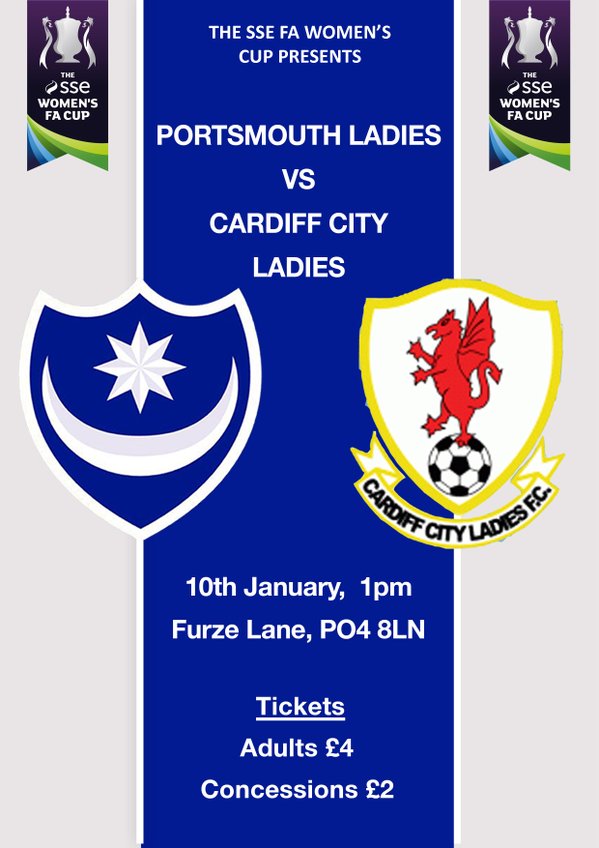The promotional poster for the SSE FA Women’s Cup features a vertical blue banner at its center with the tournament's title "The SSE FA Women’s Cup presents Portsmouth Ladies vs. Cardiff City Ladies" in white text at the top. Flanking the blue banner are grey vertical banners displaying a silver trophy beside the SSE Women’s FA Cup logo. Central to the design, the left side showcases the Portsmouth Ladies' shield, which has a white border, a blue background, an 8-point white star, and a crescent moon resembling a smile. On the right is the Cardiff City Ladies' shield outlined in yellow, depicting a red dragon balancing on a black and white soccer ball, with a yellow ribbon below reading "Cardiff City Ladies FC." Below the shields, the poster details the match specifics: "10th January, 1 p.m., Ferser Lane, PO4 8LN," stated in yellow text, followed by ticket prices: "Adults £4, Concessions £2."